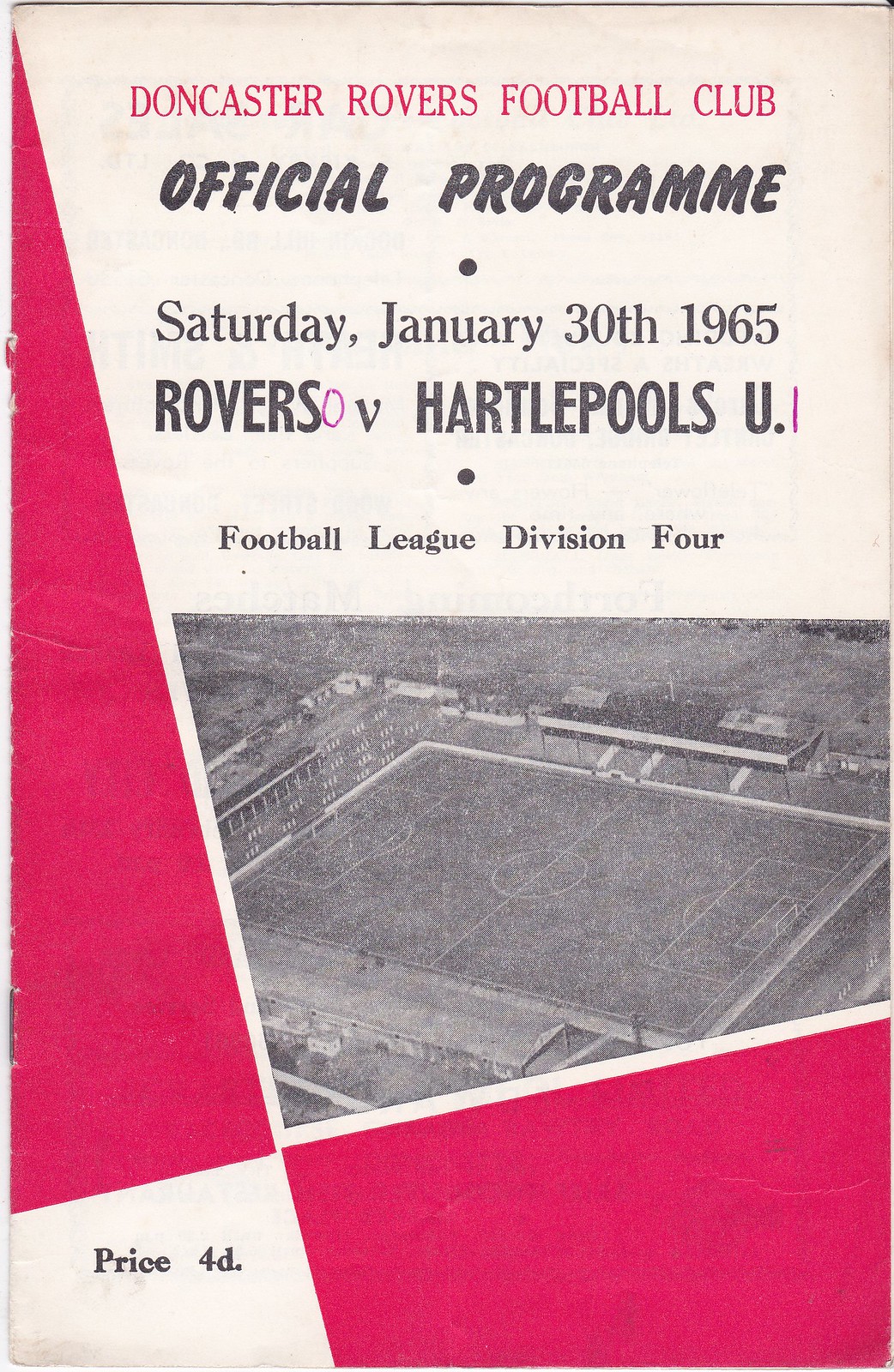This image appears to be an official game day program from the Doncaster Rovers Football Club dating back to Saturday, January 30, 1965. The design is distinctly vintage, adding to its nostalgic charm. The overall background is white, featuring red and black lettering. Dominating the top center of the cover, in striking red capital letters, is the title "DONCASTER ROVERS FOOTBALL CLUB." Just below it, in black letters, “Official Program” is printed. Underneath, the date "Saturday, January 30, 1965," is prominently displayed followed by the fixture "Rovers vs. Hartlepools U." in sans serif font. Further down, it reads "Football League Division 4" in smaller serif font.

The left side of the cover is accentuated by a long red triangle, while the bottom right-hand corner features a red square, creating a visually appealing layout. At the center of the cover is a grainy black-and-white aerial photograph of an empty soccer stadium. The bottom left-hand corner of the cover lists the price, "Price 4D," in black font. The cover shows signs of wear and staining, consistent with its age, enhancing its old-fashioned appearance.